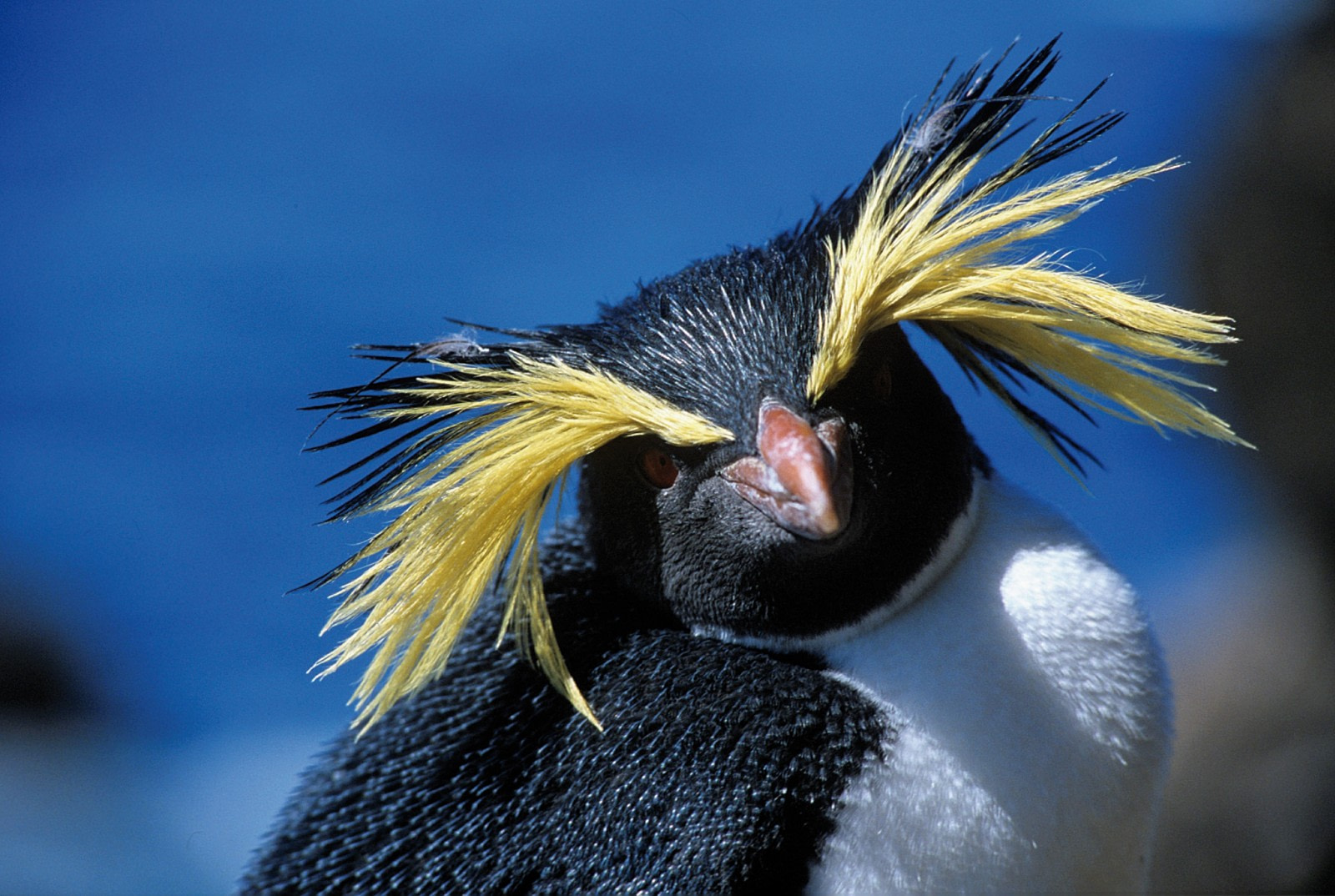This is a detailed close-up photograph of a brightly colored penguin, primarily featuring its upper torso and head. The penguin is centrally positioned against a mostly blue, out-of-focus background with some darker shadows. Its striking features include a predominantly black head adorned with long, vibrant yellow and black feathers that extend from just above its eyes and nearly touch its back and chest. The penguin's expressive brownish or reddish eyes are turned toward the camera, giving an impression of curiosity. The bird’s thick black plumage covers its back, while its front is white, complementing its orange, red, and black beak. The penguin’s overall posture has its chest facing to the right and its back to the left, with its head turned to engage directly with the camera.